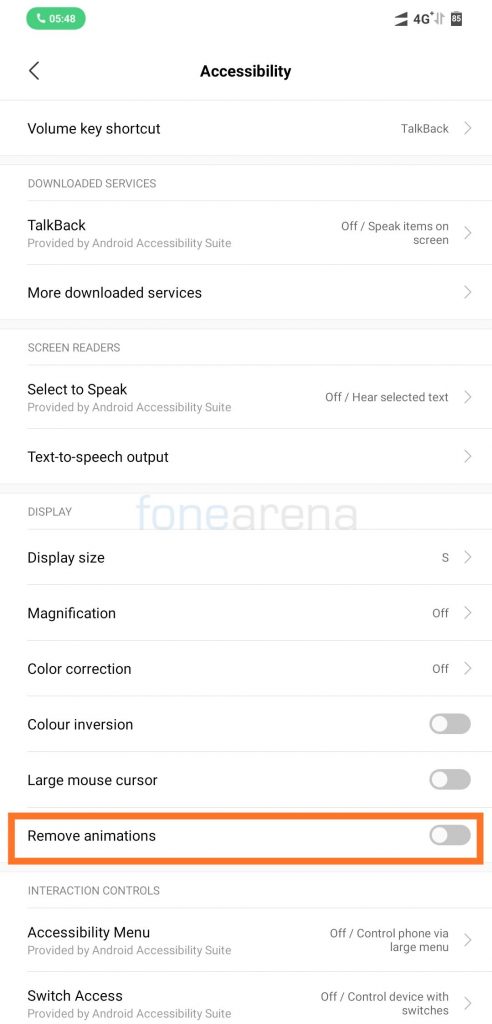This image depicts the control settings screen on a smartphone, featuring accessibility options. At the very top, a status bar indicates an ongoing phone call lasting 5 minutes and 48 seconds, displayed within a green oval in white font. Beside it, there are various phone icons including an unknown symbol, a 4G indicator, and a battery icon showing its current charge level.

The main section of the screen displays the "Accessibility" menu, prominently bolded and centered in black. To the left is a back arrow, separated by a line from the rest of the menu options. First, it lists "Volume key shortcut" with "TalkBack" indicated on the right, separated by another line. Below that, in a grayish color, is "Downloaded services," separated by another line followed by "TalkBack" provided by the "Android Accessibility Suite," with an option to toggle 'Off' or 'On' for this feature.

Further options include "More downloaded services" with an accompanying arrow indicating additional settings. Below is "Screen readers," under which "Select-to-Speak" is noted as provided by the Android Accessibility Suite, with the feature currently toggled 'Off.'

Under "Screen readers," there is a section for "Text-to-speech output," followed by various display settings. These include "Font size" (displayed in a very large font), "Display size," "Magnification," "Color correction," "Color inversion," "Large mouse cursor," and "Remove animations," each within a large square box to the left, with options currently toggled 'Off.'

Overall, the screen provides detailed control options for accessibility features on the smartphone, ensuring that users can customize their device's display and interaction methods to suit their needs.